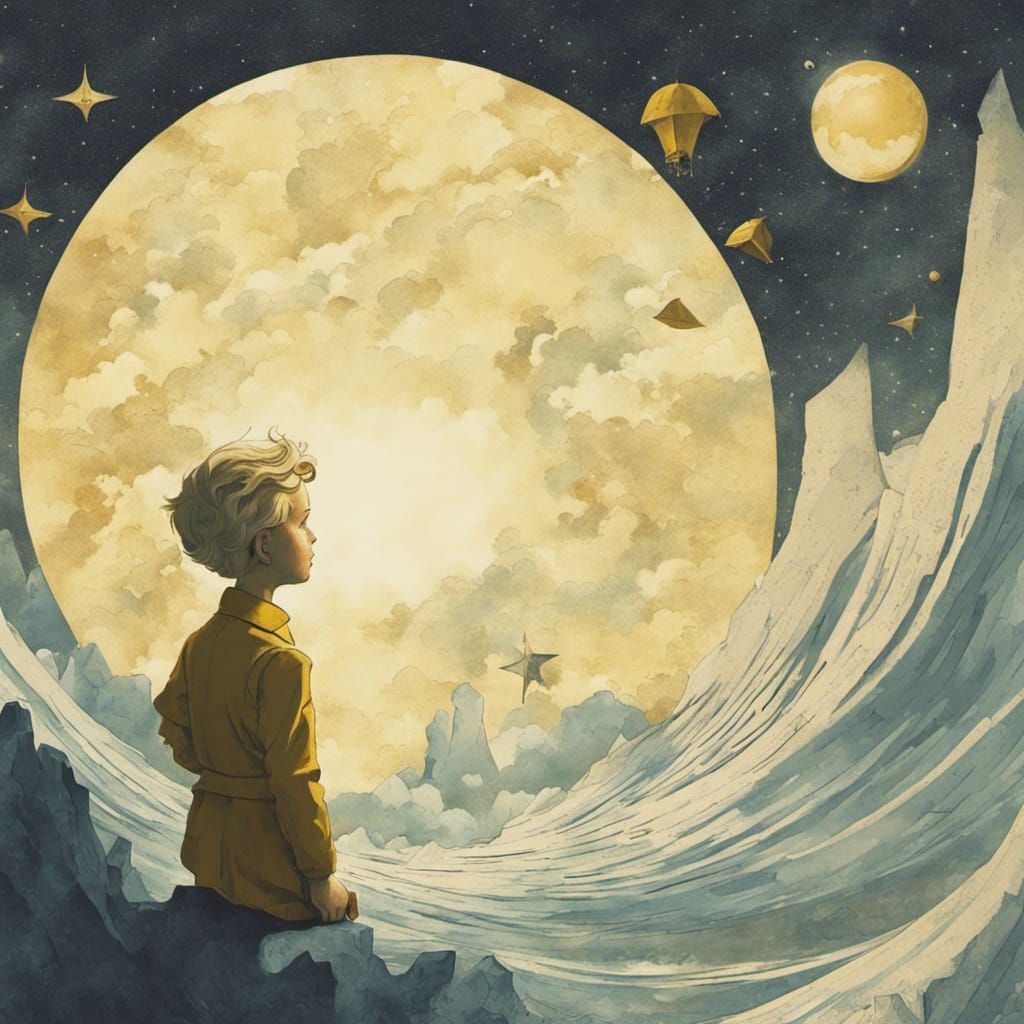This whimsical illustration, reminiscent of a classic children's book, depicts a young boy seated on jagged gray rocks in a valley. The boy, characterized by his belted yellow jacket and wavy blonde hair, gazes toward a sky inhabited by celestial wonders. Dominating the right side of the artwork is an enormous, intricately textured moon with warm hues of gold, yellow, and gray. To his left, a smaller, ecru-colored planet hovers in the dark, starlit night sky painted in deep indigos and sweeping blacks.

In the backdrop, towering white and blue mountains rise into a sky dotted with numerous bright stars. Above the mountains, a peculiar golden machine floats, resembling a hot air balloon or a tent. The dreamlike scene evokes a sense of wonder and adventure, as the boy's profile suggests he is lost in contemplation of the universe's vast expanse around him.